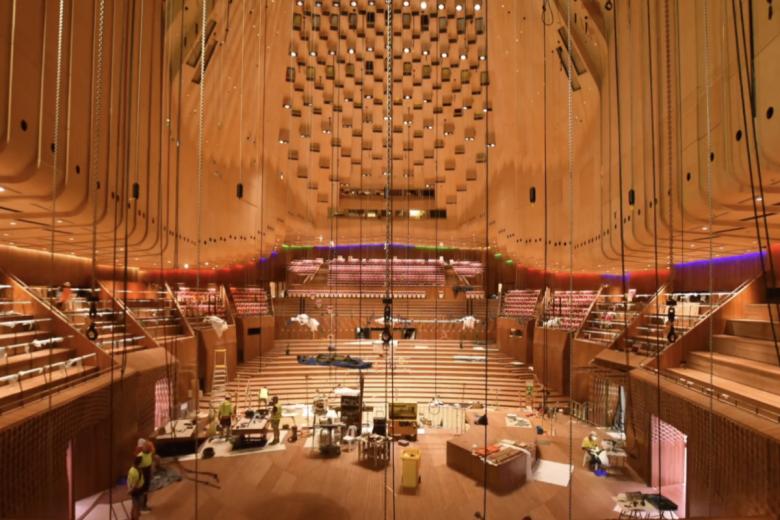The image depicts an expansive, all-wooden opera house or concert hall under construction or in the process of being set up. The arena is cylindrical in design with multiple rows and sections of seating that seem to be integrated into the structure. The focal point of the image is a large assortment of lights, many of which hang from the ceiling, extending from top to bottom. The edges of the auditorium are adorned with lights in vibrant hues of yellow, red, blue, and green. Below the main seating area, numerous workers in yellow shirts and black pants are actively moving about, setting up various instruments on numerous tables scattered across the floor. The photograph appears to be taken from behind the stage, providing a clear view of the elaborate pulley system, designed to manage the stage equipment.